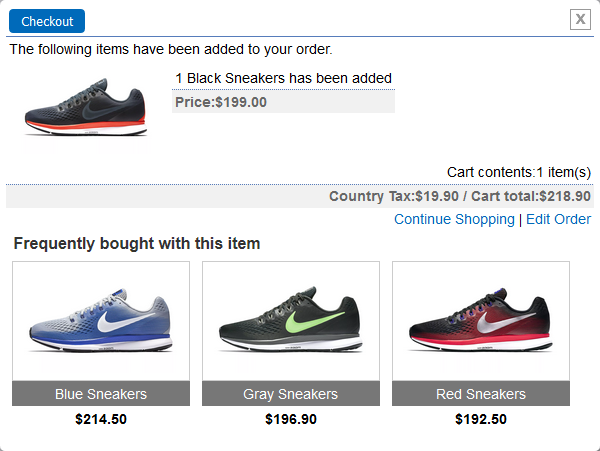The image depicts a shopping cart on an online checkout page with a clean, white background. In the top left corner, there's a blue horizontal bubble with white font text. To the right of this bubble, there is a gray square containing a gray 'X'. Below the bubble, a horizontal blue line extends from the "Checkout" label on the left to the 'X' on the right.

Prominently displayed in the cart is a Nike shoe. The shoe has a black upper part and a sole that is red-orange with a white bottom. This black sneaker is marked with a price of $1.99, which is showcased in bold font inside a light gray box. 

Below the shoe's image and price, the page lists the total number of items in the cart, the country tax, and the cart total. Options to "Continue Shopping" and "Edit Order" are provided as blue hyperlinks.

At the bottom of the page, there are three additional shoes displayed side by side. The shoes are similar in design but differ in color: a blue sneaker on the left, a gray sneaker in the middle, and a red sneaker on the right.